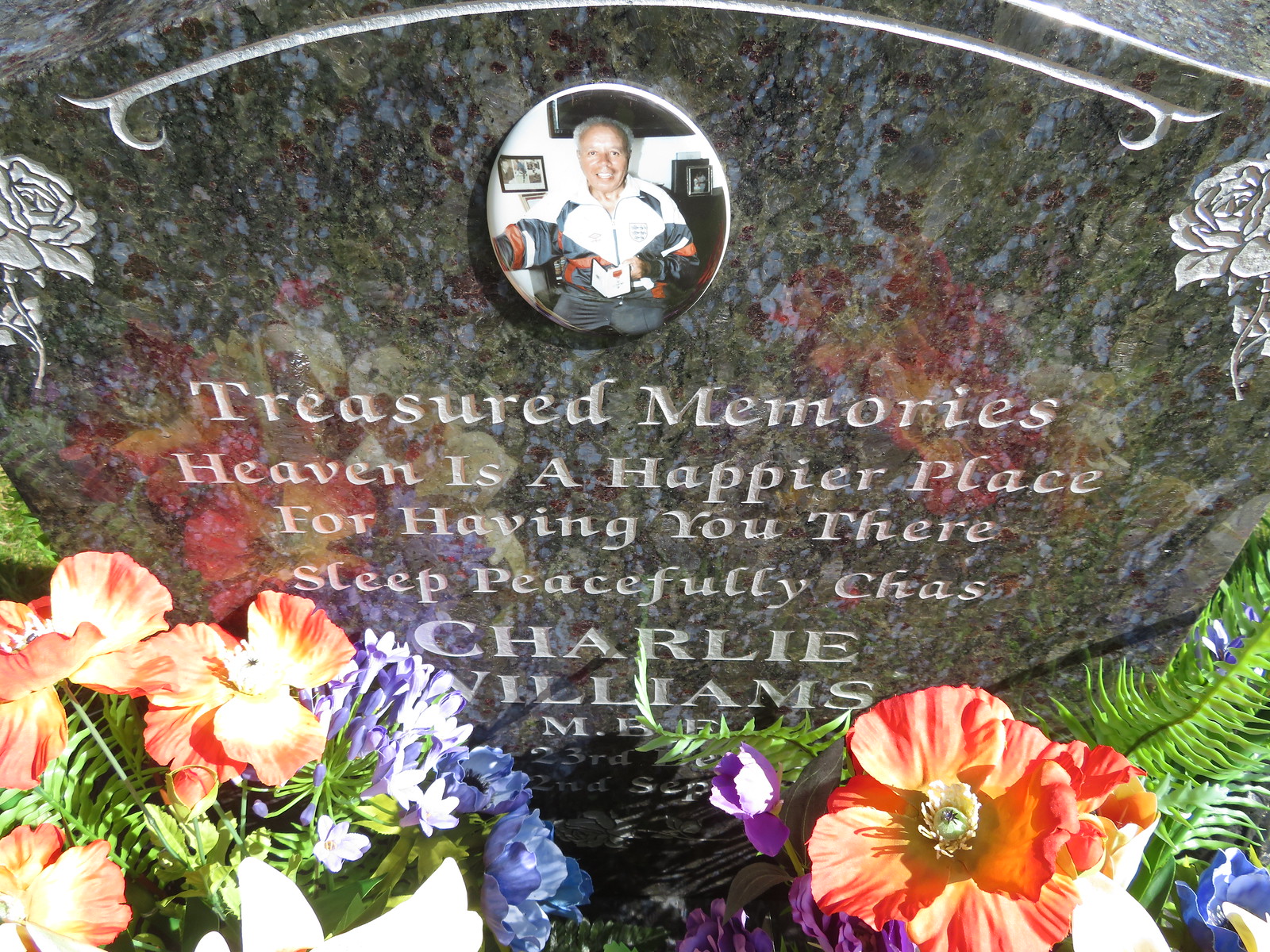The image depicts a finely crafted black marble tombstone adorned with a circular portrait of a man, who appears to be a middle-aged Black or Latino male, smiling and dressed in a black, white, and red jogging outfit. Above the portrait, two intricately engraved roses are positioned on either side. The epitaph reads: "Treasured memories. Heaven is a happier place for having you there. Sleep peacefully, Chaz." Below this heartfelt inscription, the name "Charlie Williams" is engraved. Surrounding the tombstone are vibrant bouquets of fresh flowers in colors like orange, purple, blue, and white, complemented by the lush green foliage of ferns and other plants, creating a serene and beautiful memorial setting.